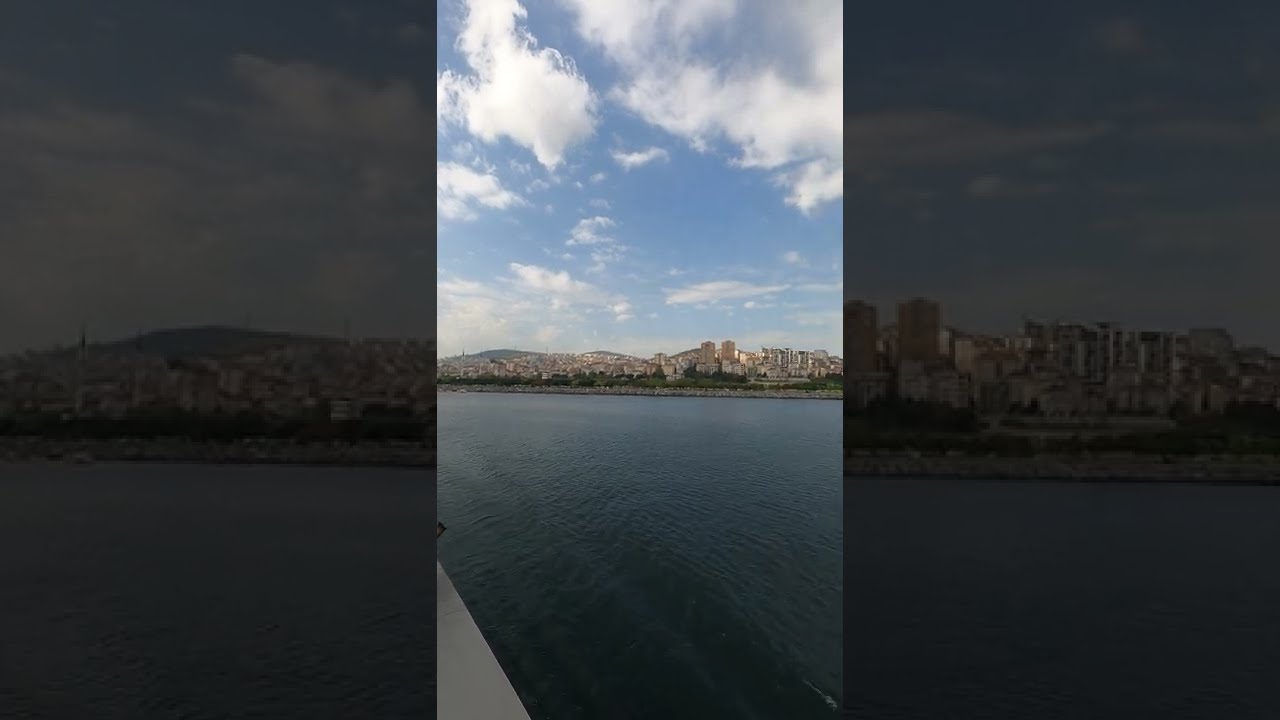The photograph, taken on a partly cloudy day, captures a scenic view of a large canal. In the foreground, a white concrete structure on the bottom left could be either a wall or a sidewalk. Opposite this, on the other side of the canal, stands a rock wall adorned with green shrubs and small trees. Beyond this greenery, a bustling cityscape emerges, with towering skyscrapers predominantly on the right and smaller buildings to the left. The water in the canal appears dark and shadowed, creating a stark contrast to the varied textures and colors around it. The sky above is scattered with puffy, white clouds, adding depth to the scene. No people or text are present in this serene cityscape, which centers on the interplay of natural and urban elements.